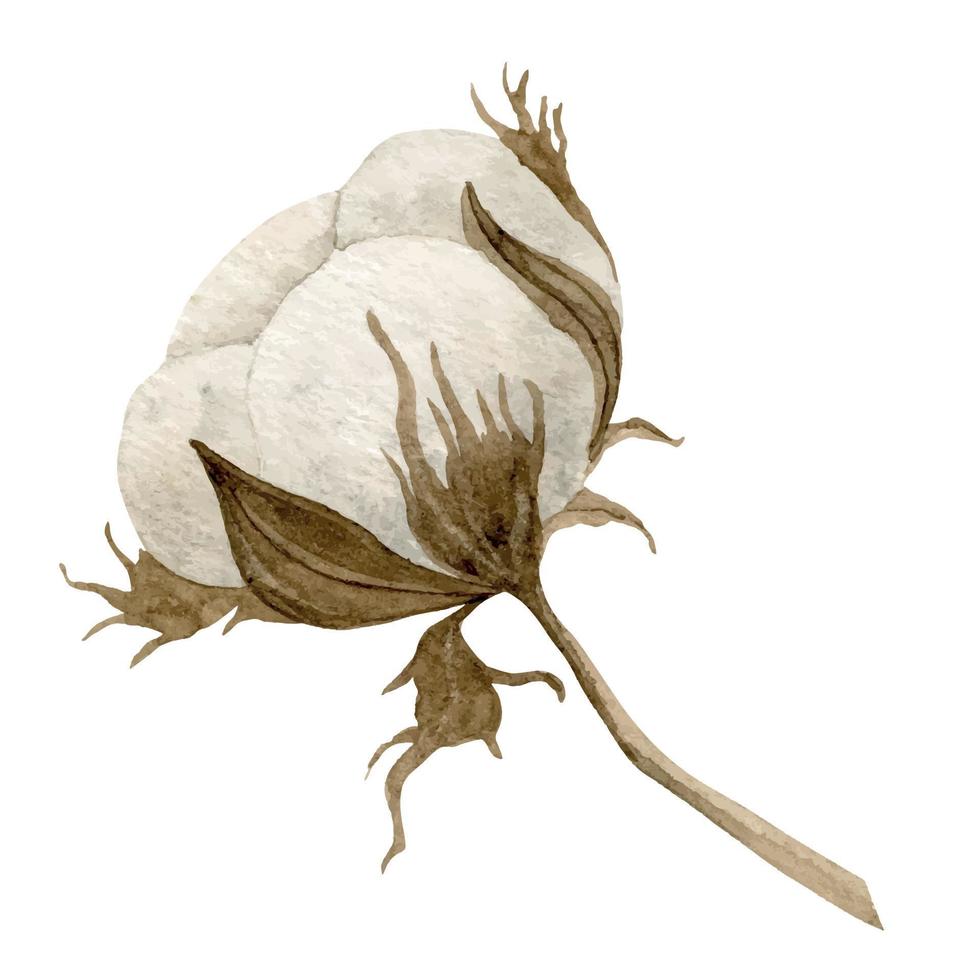The illustration depicts what appears to be a cotton plant, characterized by its brown stem adorned with a few withered-looking leaves wrapping around the soft, white cotton fruit. The cotton itself is depicted with a wispy texture and segmented into four distinct parts, giving it a fluffy, almost dough-like appearance. The brown stem rises from the bottom right to the top left of the image, contributing to the visual flow. The background is entirely white, providing no additional context and making the creamy white cotton and brown stem and leaves stand out against this stark backdrop. The overall style of the image is painterly, with a focus on the texture and segmented structure of the cotton fruit.